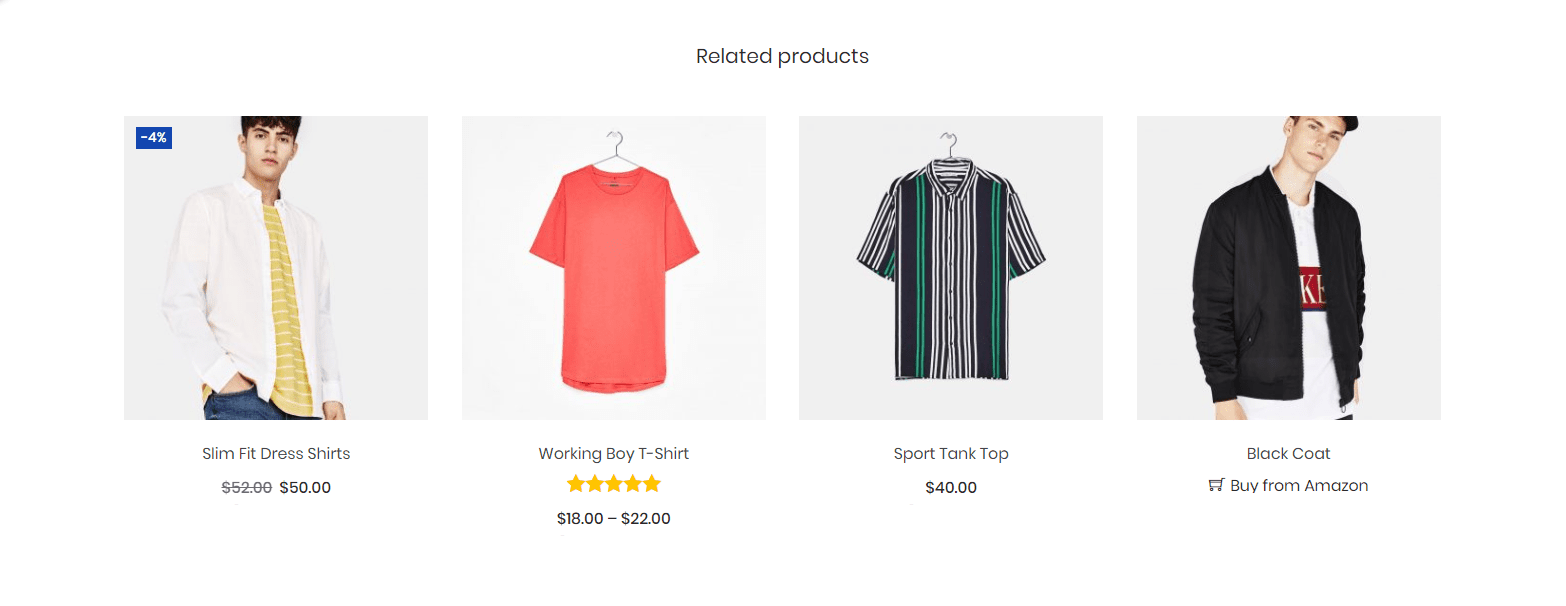This image is divided into four distinct square sections, each showcasing a different product under the header "Related Products."

- **First Square:** Features a Caucasian male wearing a long-sleeve white button-down shirt, which is unbuttoned. His right hand is tucked into his blue jean pants pocket, and underneath the white shirt, he wears a gold and white striped shirt. In the upper left corner of this square, there is a label indicating a 4% discount. Below the image, the text reads "Slim Fit Dress Shirts," originally priced at $52, now on sale for $50.

- **Second Square:** Showcases a "Working Boy T-Shirt" in a pinkish-peach color. This shirt has received a perfect rating of five stars out of five, indicating high customer satisfaction. The price range for this t-shirt is between $18 and $22.

- **Third Square:** Displays a "Sport Tank Top" priced at $40. No additional details or ratings are provided for this item.

- **Fourth Square:** Features a black coat that can be purchased from Amazon. No price or further details are mentioned, highlighting just the product and its availability on Amazon.

This detailed layout offers insight into various related apparel items, complete with pricing, discounts, and customer ratings where available.